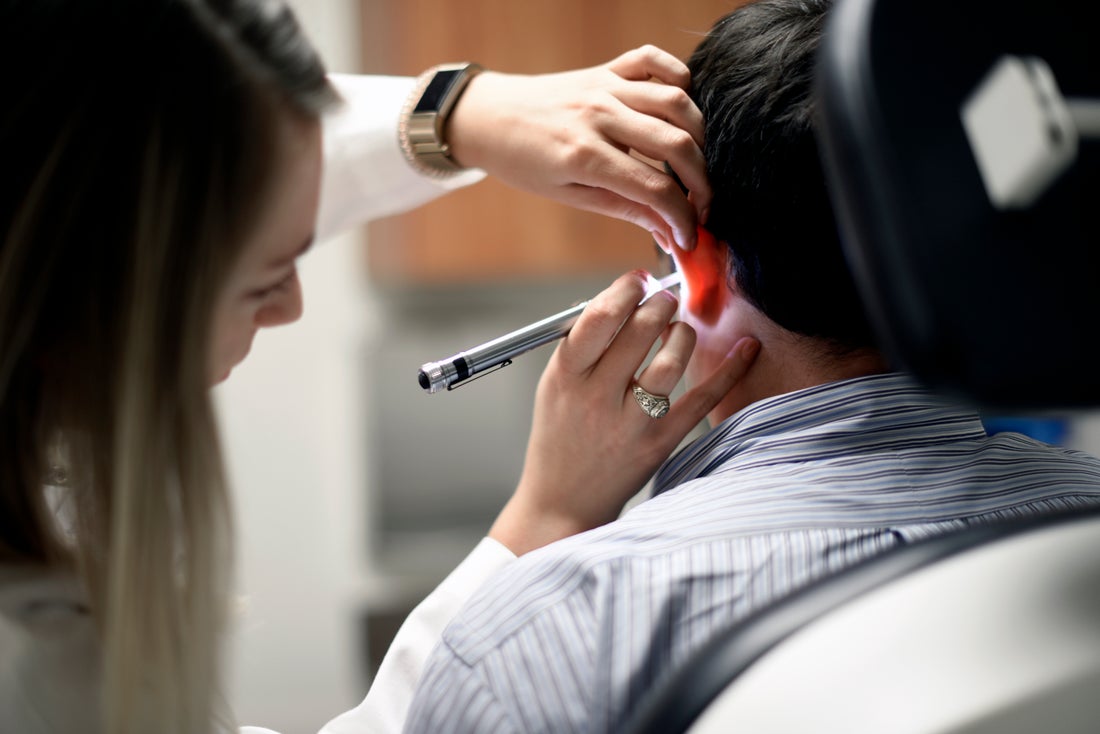The image is a detailed color photograph in landscape orientation, depicting a female doctor performing an ear examination on a male patient in a medical facility. The patient, seated in a specialized medical chair on the right side of the image, is facing away from the viewer. He has short black hair and is wearing a collared shirt with light and dark blue stripes. The doctor, positioned on the left, is leaning toward the center of the image, intently examining the patient's left ear. She has long hair that transitions from a dark color at the top to a lighter blonde at the bottom and is wearing a white lab coat. Her left hand holds the patient's ear lobe, while her right hand steadies a glowing pen light inside the ear. She is adorned with a ring on her right ring finger and a gold watch on her left wrist. Behind the doctor, parts of the medical office, including a counter and cabinets, are visible but out of focus. The composition captures the professionalism and meticulousness typical of healthcare environments.